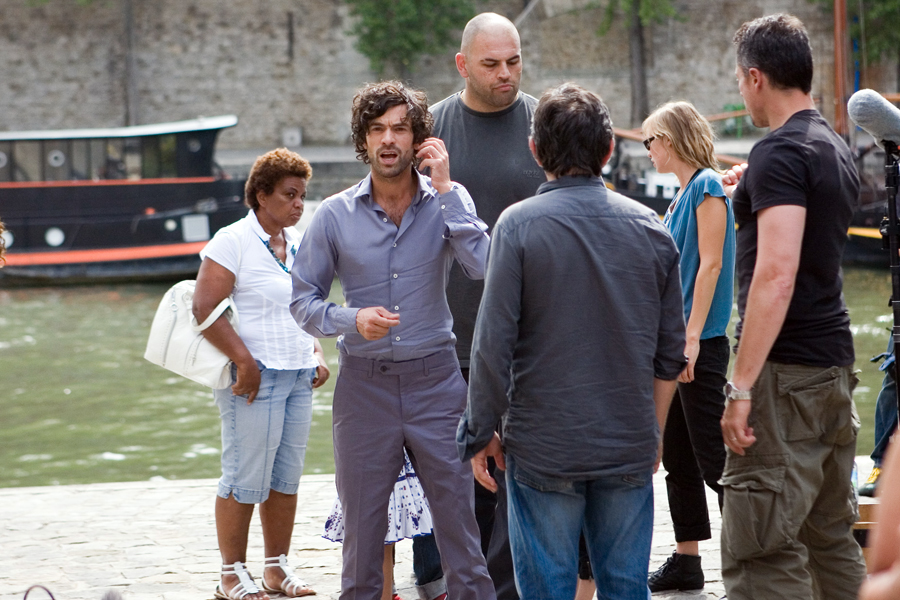A lively scene unfolds at a concrete pier with serene waters serving as a backdrop. In the distance, a small tour boat is anchored, ready for its next adventure. The foreground is bustling with a group of five to six people, all casually dressed, seemingly waiting for the arrival of a boat. 

One individual stands out, dressed in dark gray pants and a light gray, open-collared shirt. He appears to be holding a cell phone in his left hand, which is positioned to the right in the photo. His features are distinct, with very curly hair and a light mustache and beard.

Next to him is a tall gentleman with a bald head, donning a dark gray t-shirt. Beside him stands a blonde woman in a turquoise, sleeved blouse paired with dark pants. She is noticeable for her short boots, and although she seems to have no visible socks, it adds a casual, laid-back vibe to her ensemble. The scene captures a moment of anticipation and tranquility, set against the picturesque backdrop of the pier.